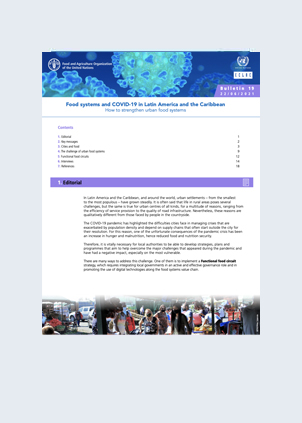This image features a graphical, text-based, PDF-style document resembling a poster or advertisement, likely part of a larger publication. The displayed page appears to be a contents or editorial page, cut and pasted onto a plain grey background. Due to the low image quality, both the text and visuals are quite blurry. The header section is adorned with stylized graphics resembling viruses or bacteria, rendered in blue and green hues. The title of the document, though difficult to read, is in blue text and reads "Food Systems and COVID-19 in Latin America and the Caribbean: How to Strengthen Urban Food Systems." The contents menu lists sections and their corresponding pages. The main content of this page features an editorial block of text alongside a summary. At the bottom, there are images depicting groups of people, possibly at food banks or similar community food distribution events.